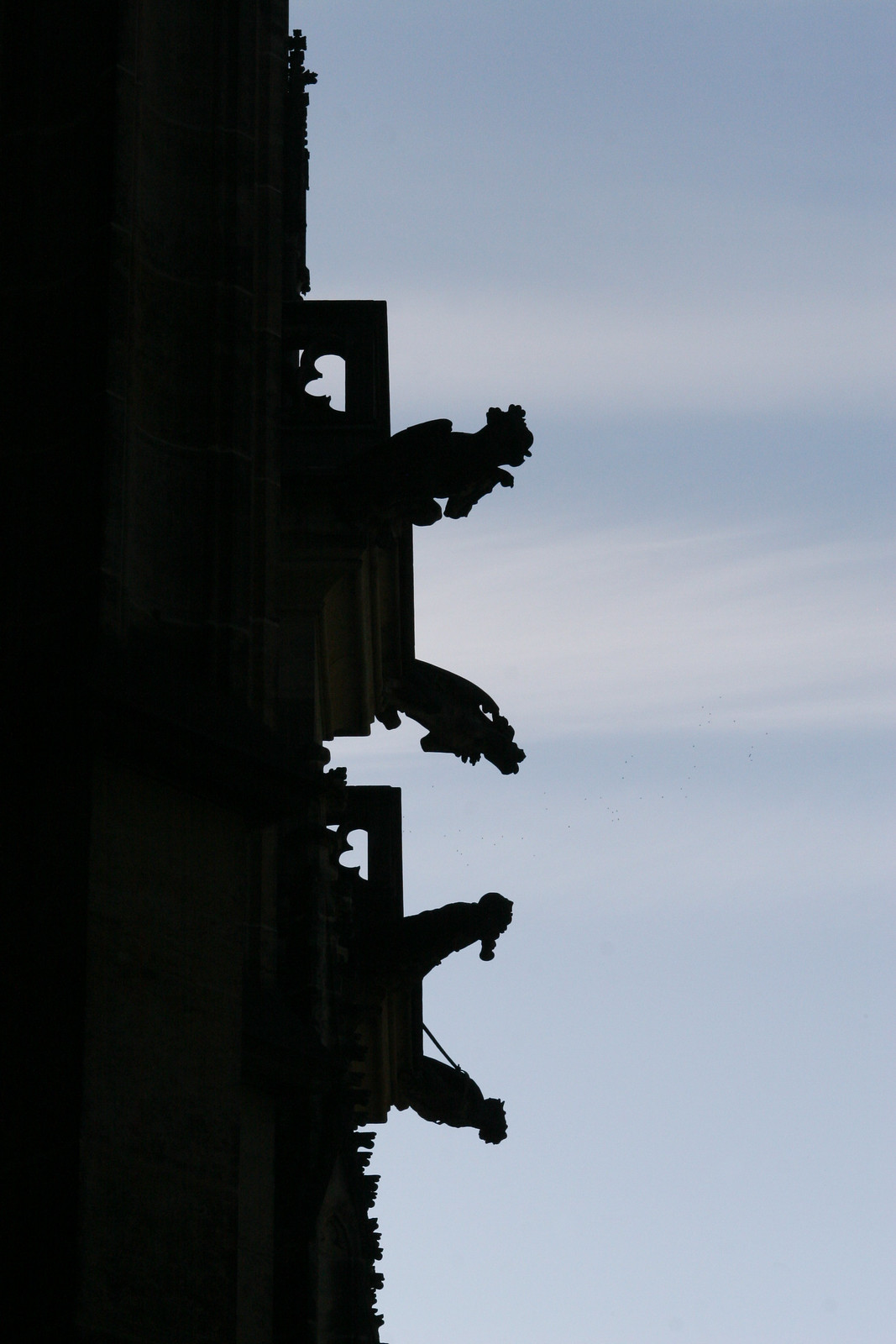The photograph appears to be turned 90 degrees to the right, presenting an outdoor scene with a striking contrast between the sky and a silhouette. On the right side of the image, a vibrant blue sky is streaked with white cirrus clouds, resembling artistic brushstrokes. The left side of the image is entirely in black silhouette, making it challenging to discern the specific objects. This dark silhouette seems to depict rampart-like structures with ornate statues at the top, potentially resembling people or creatures. Alternatively, the silhouettes could represent two oil rigs side by side with distinct shapes protruding upwards, including rectangular iron structures. The overall impression is a dramatic interplay between the detailed sky and the mysterious, shadowy forms.